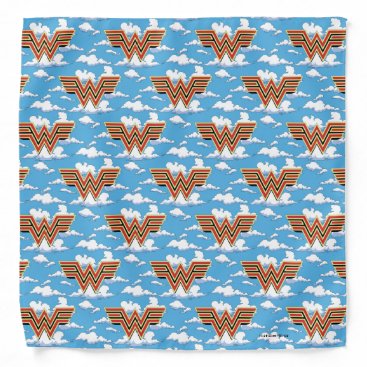The image showcases a blue sky with white clouds as a background, featuring a repeating vintage Wonder Woman logo in a distinctive pattern across the surface. Specifically, the logos form a 3-4-3-4-3 arrangement across seven rows. The logos, colored in red, black, and tan, contrast sharply with the serene sky-blue backdrop. The image, resembling a piece of textured fabric such as a quilt or fleece blanket, has a slightly lifted bottom left corner with a visible shadow underneath. While one caption mentions unreadable text near the bottom right of the image, the primary focus remains the vivid repetition of the Wonder Woman emblem against the cloud-studded sky, making it ideal for wallpaper or other decorative purposes.